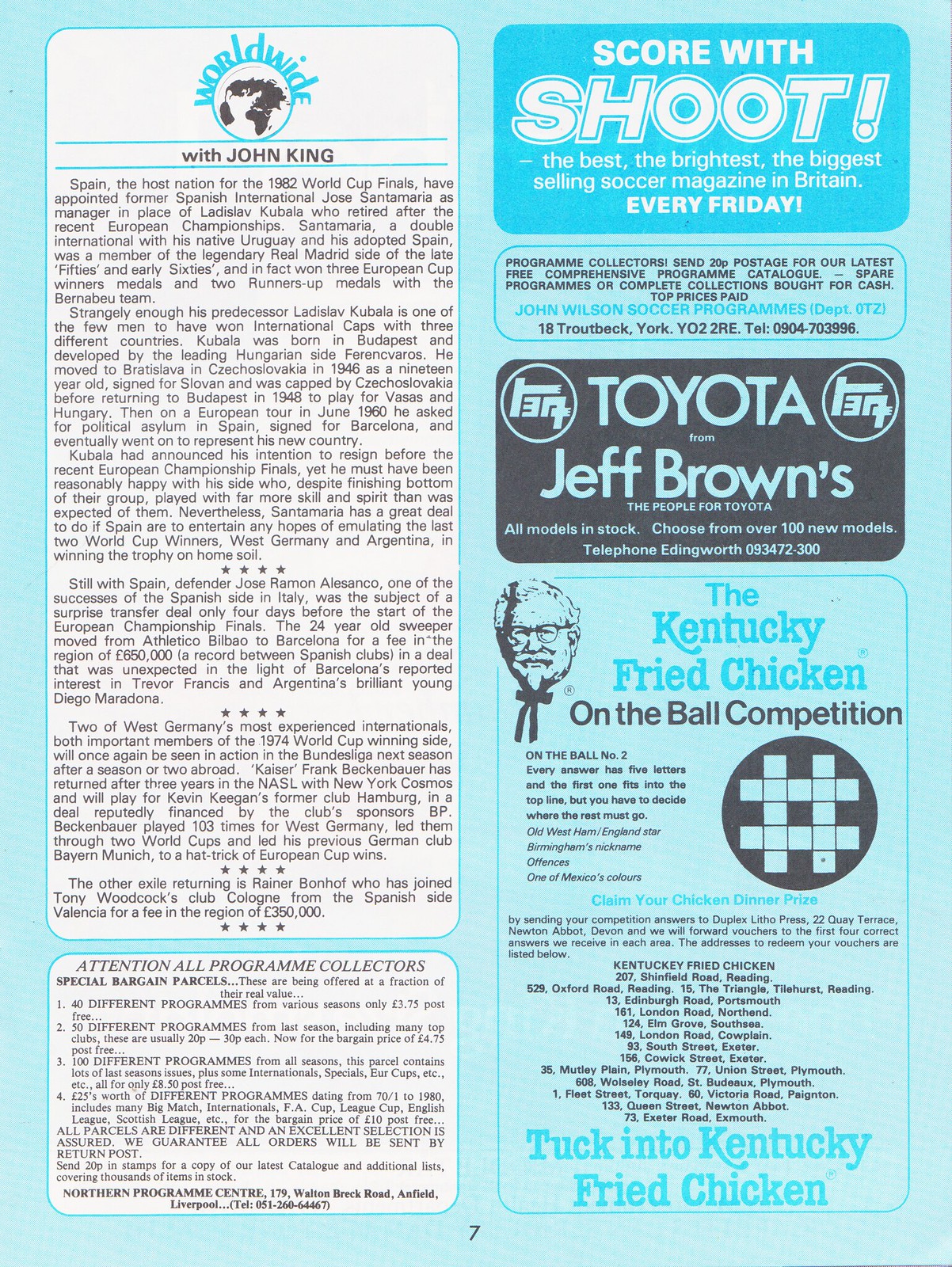This vintage newspaper advertisement has a light blue background with various sections promoting different products and services. In the upper right corner, a blue square prominently features the text: "Score with Shoot – The Best and Brightest, the biggest selling soccer magazine in Britain, every Friday." Below this, an advertisement caters to program collectors, inviting them to send £20 postage for a "free comprehensive program catalog" from John Wilson Soccer Programs, Department 0721. Next, there is a black square promoting "Toyota, from Jeff Browns," highlighting a selection of over 100 new Toyota models with a corresponding telephone number. Further down, an ad features "The Kentucky Fried Chicken On The Ball Competition," adjacent to Colonel Sanders' logo, with information at the bottom encouraging readers to "tuck into Kentucky Fried Chicken" and listing several locations. On the left side of the page, a white rectangle houses an extensive article titled "Worldwide with John King," accompanied by a black and white globe illustration, followed by two paragraphs under the header "Attention all program collectors," discussing special bargain parcels of various soccer programs.